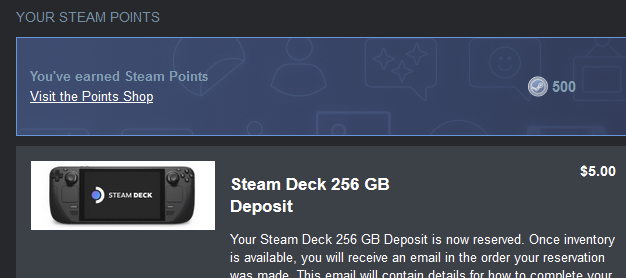The image features a sleek, dark-themed interface with various design elements and text. At the top, there's a black background overlaid with light blue font, accented by a blue-outlined box with a blue background on the left. Inside this box, it reads "Your Steam Points" in a bold blue font, followed by the text "You've Earned Steam Points" in a different shade of blue. Below this, in underlined white font, is the call-to-action "Visit the Point Shop."

To the right of this section is a gray circle containing a white image, flanked by the number "500" in a grayish-blue font. Adjacent to this are a series of icons, including a depiction of a person’s head and shoulders, a half circle to the left, a blue square with three stars, another square featuring a happy face, and yet another square with a briefcase handle design.

At the bottom left, on a grayish background, there’s a white box housing the image of a gray-colored device with handles on either side. Centrally positioned within this box, in white font, is the text "Steam Dock" accompanied by a blue circle and a partially white circle. To the right of this box, in white font, it states "Steam Deck 256 GB Deposit" with the price " $5 " nearby. Beneath this, also in white font, is a message that reads: "Your Steam Deck 256 GB Deposit is now reserved. Once inventory is available you will receive an email in the order your reservation was made. The email will contain details for how to complete your reservation."